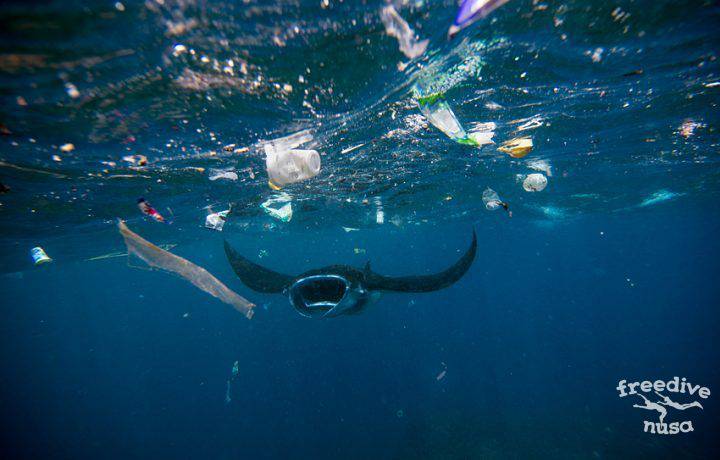This color underwater photograph captures a large, majestic manta ray swimming towards the photographer with its mouth wide open. The setting is near the surface of a traditional blue ocean, where light filters down through the rippling waves. The water is heavily polluted, with a variety of debris including plastic cups, bottles, and other trash both floating at the surface and sinking below. The distressing state of the water suggests an urgent need to address ocean pollution to protect marine life. In the bottom right corner, there is a white logo that reads "Free Dive Nusa," flanked by silhouettes of two divers.